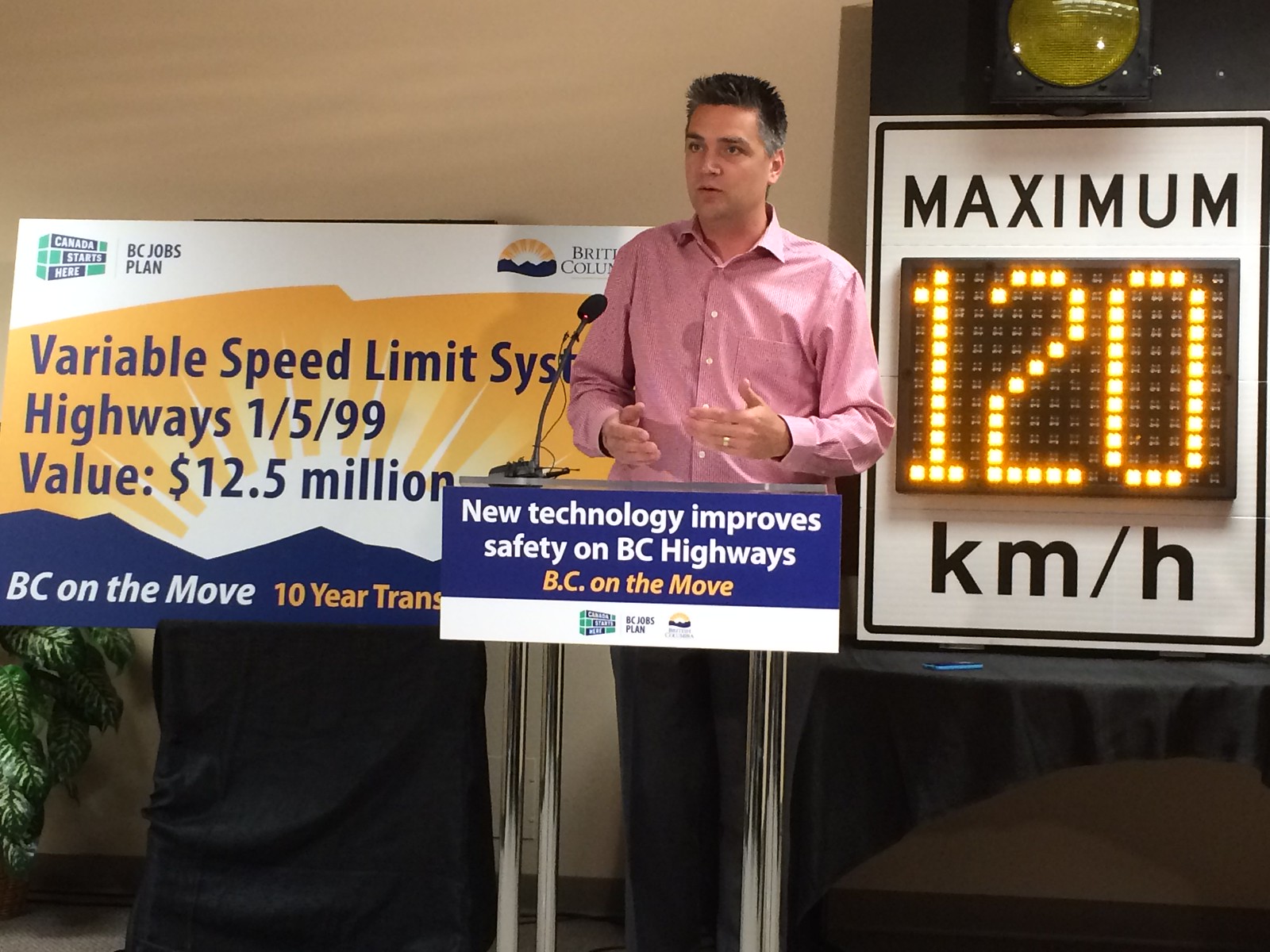In this detailed color photograph, we see an indoor setting with a man, likely in his 30s or 40s, standing at a podium and speaking to an unseen audience. The man, a white individual with short black hair featuring some gray strands, is dressed in a long-sleeve pink shirt and dark pants. His hands are raised in front of his chest as he gestures during his speech, and a black microphone extends from the left side of the podium.

The podium itself bears a prominent blue rectangle with white and yellow text that reads, "New technology improves safety on BC highways." Directly beneath this, in yellow text, it states, "BC on the move," accompanied by a white strip featuring several sponsor logos, including one that says "Canada starts here." Behind the man, on the left side of the image, there is a horizontal poster with a white heading displaying logos and the text "Variable Speed Limit System, Highways 1 / 5 / 99, Value: 12.5 million" against a gold background with a white rising sun graphic. 

To the right of him is a road sign indicating the maximum speed limit, "Maximum 120 km/h," with the digits shown in a lit-up yellow display. The background includes a beige wall adorned with an ornamental plant at the lower left corner and a table covered with a black cloth, holding a cell phone or pen. This event, seemingly a hosted meeting, focuses on the introduction of new technologies aimed at improving highway safety in British Columbia, as highlighted by the detailed signage and informational graphics present in the scene.